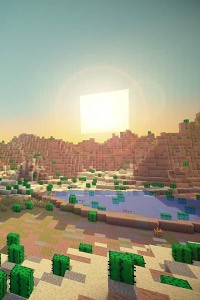In this small, pixelated image reminiscent of a classic computer game, the foreground features a cement walkway composed of little green squares. The walkway presents a gradient, with a light tan hue on the right transitioning to a darker tan on the left. Central to the scene is a body of water shaped like a triangle, creating a focal point amidst the pixelated terrain. Beyond the water, the landscape extends into mountainous formations, adding a sense of depth and adventure to the pixelated world.